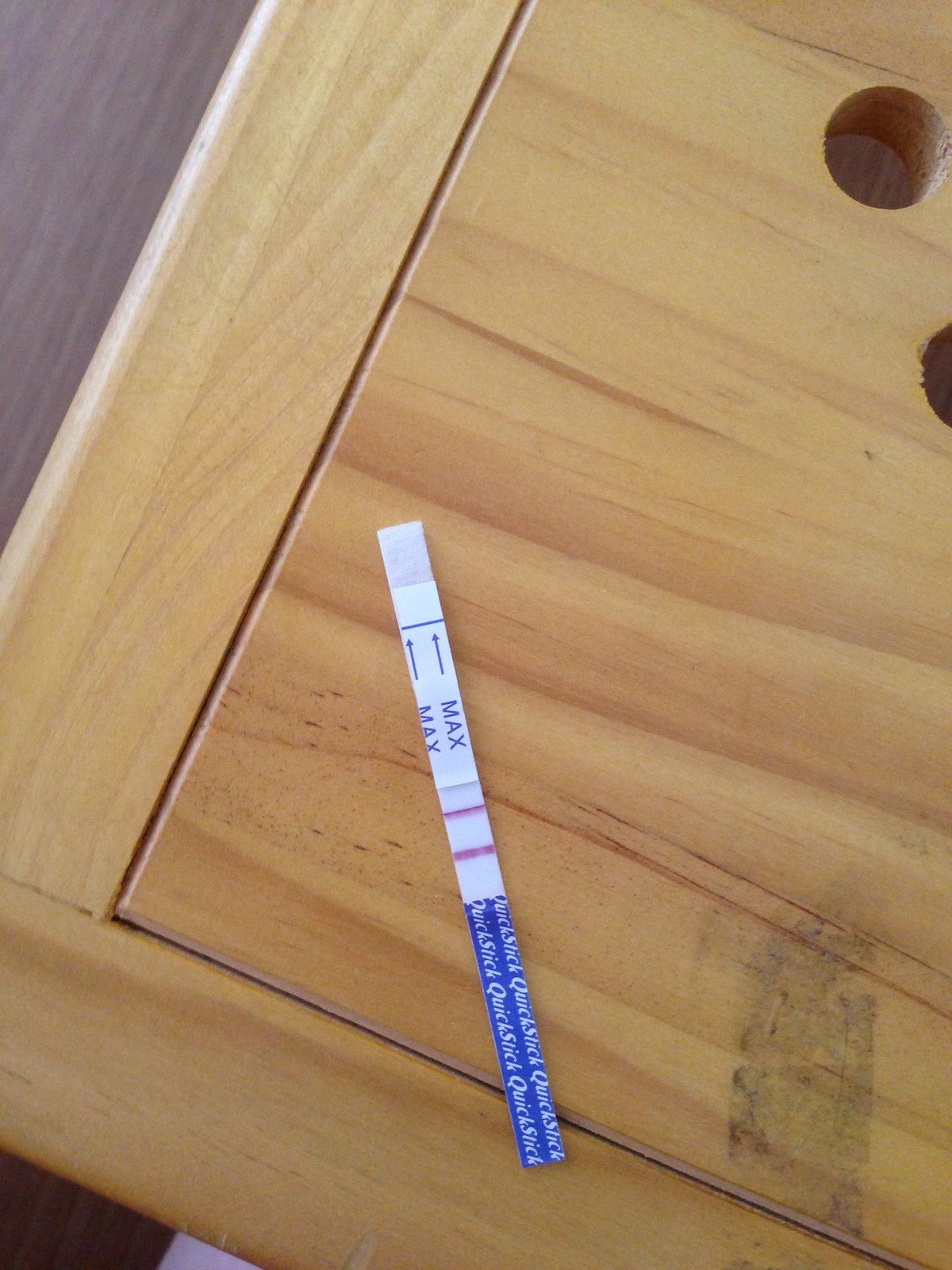This photograph captures the corner of a light blonde wood-stained table, highlighting its texture and detailing. The table shows signs of everyday use, evidenced by a complete hole and a partial, diagonal hole near the corner, as well as a distinct black scuff mark that resembles a shoe print. Resting on the table is a long, slender box, predominantly blue with "Quick Stick" written multiple times in white italic print. The upper half of the box is white, featuring two pink lines and a label marked "Max" with an upward-pointing arrow, followed by another "Max" with an additional upward-pointing arrow, indicating a pregnancy test. The table's grain pattern adds to its character, with irregular, contrasting bands ranging from light to reddish-brown shades.